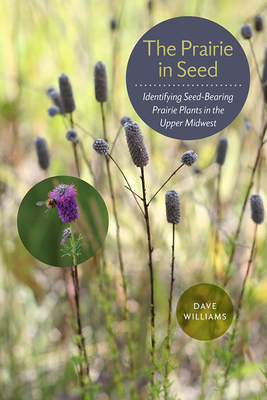This image features an in-focus, close-up photograph of seed-bearing prairie plants, framed in a portrait mode. The plants are characterized by long brown stalks with vertical oval-shaped tops, some of which are blooming. A standout bloom features a tall, narrow purple flower atop a green stem, situated on the left side of the image. The background is filled with blurred, green foliage that highlights the prominence of the plants in focus.

At the upper right-hand corner, a gray circle with yellow text reads, "The Prairie in Seed," and below it, in white text, "Identifying Seed-Bearing Prairie Plants in the Upper Midwest." This text suggests that the image serves as a cover for educational material, likely a book or magazine, focused on prairie plants.

Additionally, a small honeybee or bumblebee can be seen resting on one of the purple flowers, adding a touch of natural life to the scene. At the bottom of the image, another circle, possibly green, contains the author’s name, "Dave Williams," in white text. The overall palette of the image consists of earthy tones, primarily greens, purples, and browns, enhancing its natural springtime theme.